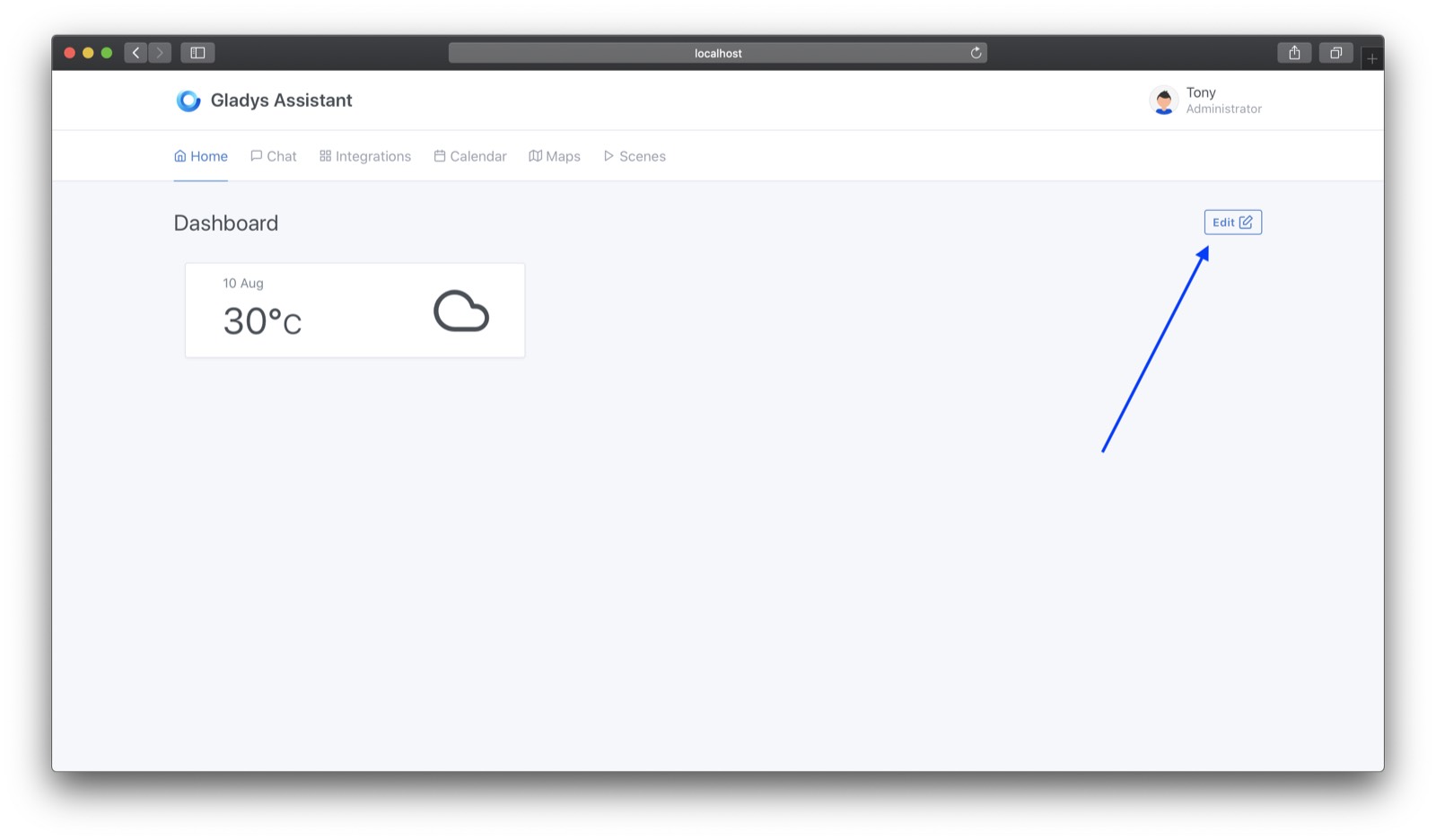The website interface depicted in the image features a light black banner at the top, which includes three colored dots on the left side—red, yellow, and green—from left to right. Adjacent to the dots are two square icons: the first one contains a left-pointing white arrow that is faintly visible, and the second, clearer arrow points to the right. Additionally, there's a rectangular icon resembling a book or calculator with varied thickness on its sides. 

Next to this icon, a gray search bar is present and it reads "localhost" alongside a refresh symbol. Adjacent to this, a square icon with an upward arrow is positioned, followed by two more square icons. Below this, the main interface extends to a clean, white page, featuring a blue circle at the top that reads "Gladys Assistant," with the initials "G" and "A" capitalized. 

On the far right, there is a circular icon with a cartoon image of a boy and the text "Tony Administrator." A row of navigation titles follows beneath the banner, listing: Home, Chat, Integrations, Calendar, Maps, and Scenes. The Home tab is highlighted in blue with an underline to indicate the current selection. 

The next section showcases a light gray background with the heading "Dashboard." Beneath this heading, a white box displays the date "10 Aug," the temperature "30°C," accompanied by a cloud icon. To the right of this, there's an upward diagonal blue arrow pointing to the word "Edit," which is enclosed in a blue square.